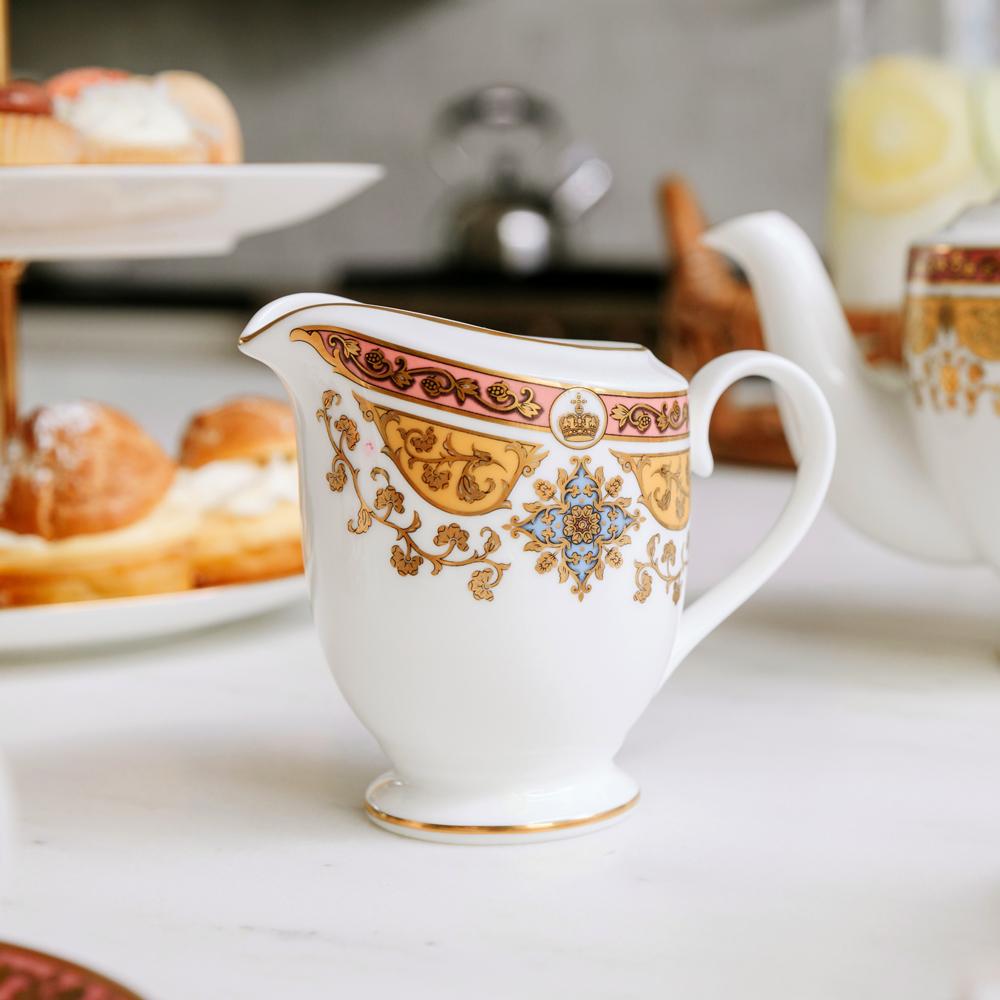This detailed image captures a tea setting elegantly arranged on a white, marble-like table. At the center is a white ceramic creamer cup with ornate decorations. The cup features a curved handle and is trimmed with gold around both the base and the rim. Its sides are adorned with a decorative pattern of pink, blue, gold, and yellow elements, including a small crown illustration above a light blue cross surrounded by gold filigree.

To the right of the creamer is a partially visible white teapot that shares a similar design, characterized by a red band at the top and gold details below. On the left, there is a two-tiered platter displaying an assortment of pastries, likely cream puffs dusted with powdered sugar. 

In the background, slightly out of focus, a silver tea kettle sits atop a stove, next to a wooden sugar bowl with a spoon sticking out. The overall scene is set against a pale gray wall, providing an understated backdrop that highlights the intricate details of the tea set.